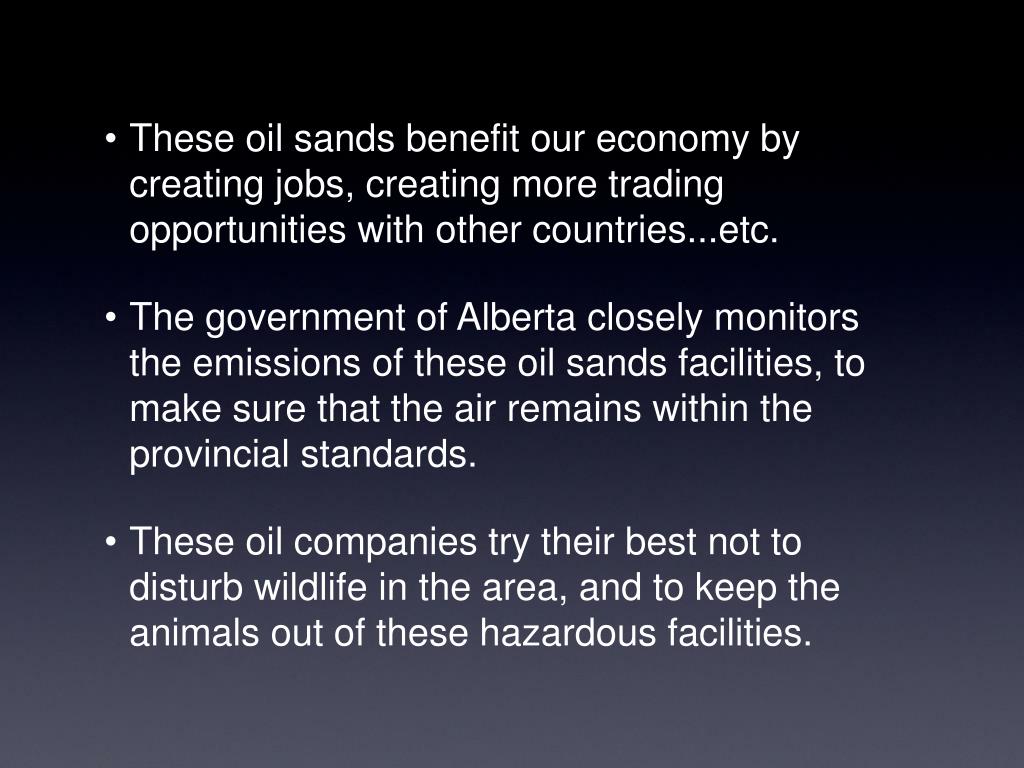The image features a gradient background that transitions from jet black at the top to a lighter charcoal gray and then fades into dark purple and light purple towards the bottom. Centered against this background are three bullet points in white sans-serif font. The first bullet point states, "These oil sands benefit our economy by creating jobs, creating more trading opportunities with other countries, etc." The second bullet point reads, "The government of Alberta closely monitors the emissions of these oil sands facilities to make sure that the air remains within the provincial standards." The third bullet point mentions, "These oil companies try their best not to disturb wildlife in the area and to keep the animals out of these hazardous facilities." The text is positioned centrally, suggesting it could be part of a book, magazine, article, or an online publication. There are no objects in the image, just the descriptive text on a richly shaded background.